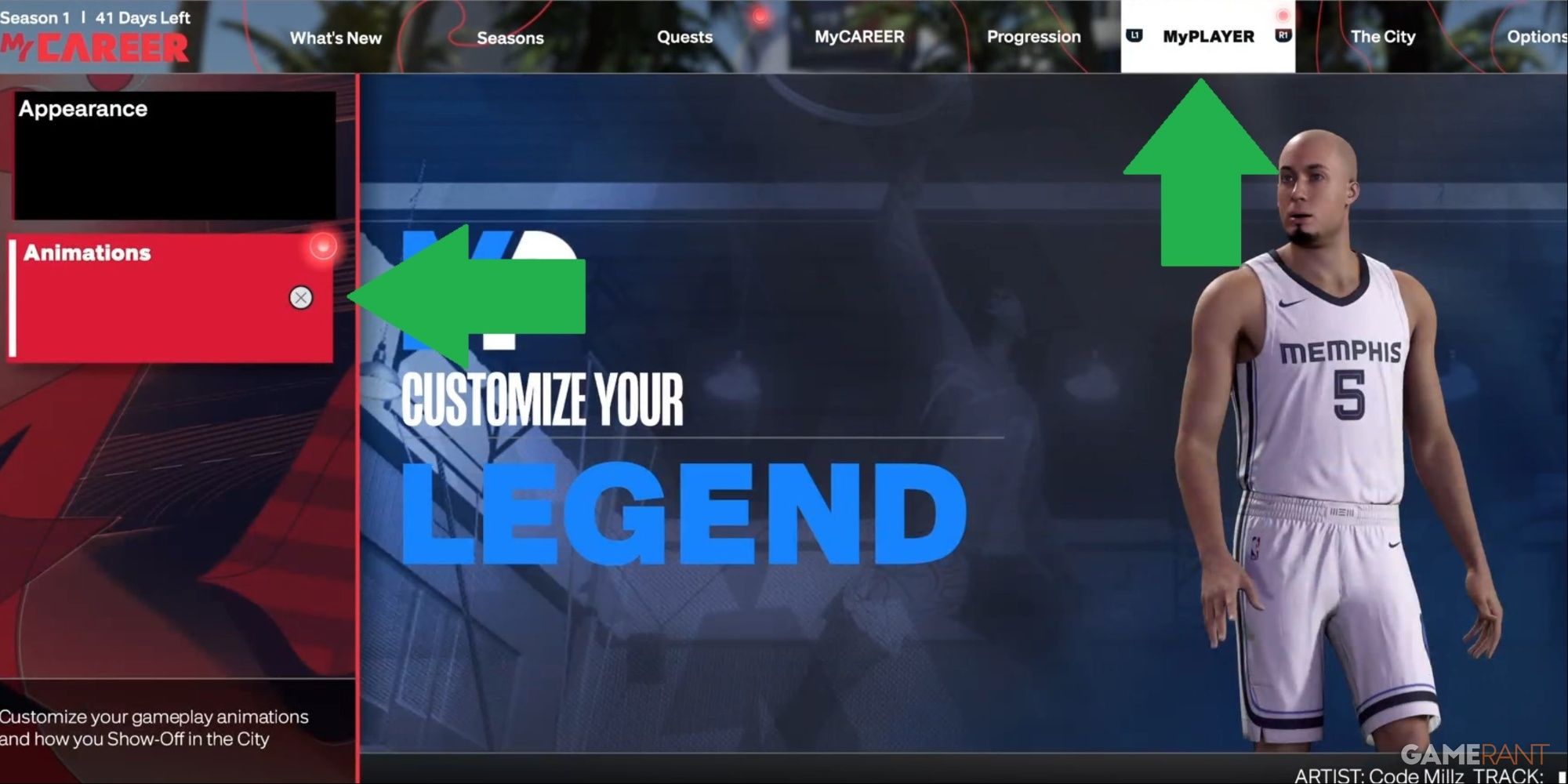In this image, you see a screenshot from a basketball video game featuring a computer-generated player. The player, sporting an all-white jersey emblazoned with "Memphis" and the number 5, is adorned with Nike logos. The player has a bald head, a beard, and is gazing to the left of the screen.

On the left side of the screen, the phrase "Customize Your Legend" is prominently displayed, accompanied by a green arrow pointing towards a red box labeled "Animations." Directly above this box is another black box labeled "Appearance." 

At the top of the screen, a menu bar featuring different categories, from left to right, reads: "What's New," "Seasons," "Quest," "My Career," "Progression," "My Player," "The City," and "Options." The "My Player" category is highlighted with a white box and another green arrow pointing at it from below. To the right of this arrow is the computer-generated basketball player.